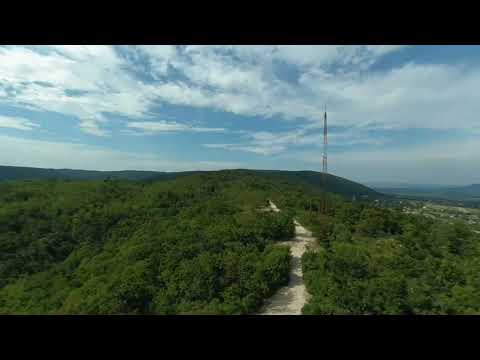This photograph captures a vast, peaceful, and lush green mountainous terrain, likely resembling something from the Appalachian Mountains. The foreground is rich with dense green treetops, among which a light sandy-colored dirt road weaves its way, creating a picturesque pathway perfect for hiking. As the view extends further, the expansive forest continues to dominate the scenery, spreading across rolling hills and giving a sense of endless greenery.

Prominently featured is a tall metal tower, painted in red and white, standing on the right side of the dirt path and piercing through the treetops. It resembles a cell phone tower or some sort of satellite structure, adding an element of human-made presence in this natural setting. The background reveals a tranquil blue sky filled with varying shades of white and gray clouds, indicating a bright and sunlit day. This setting, with its serene atmosphere and vibrant greenery, suggests a calm and inviting environment, ideal for outdoor adventures and immersion in nature. Possibly a few distant houses can be spotted, hinting at nearby civilization amidst the vast wilderness.